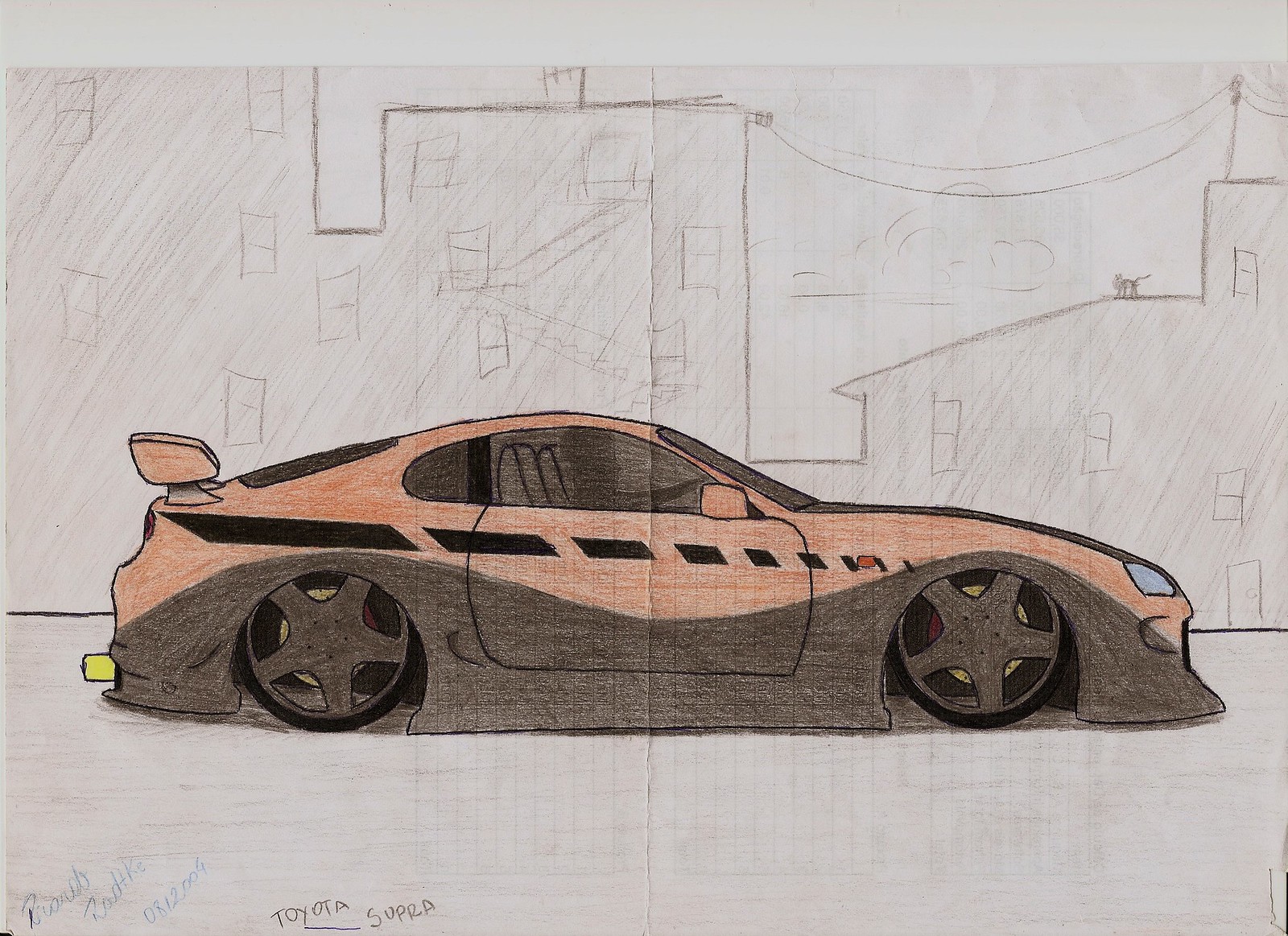This detailed sketch depicts an elegant, long, low-slung coupe, characterized by its sleek design and aerodynamic spoiler at the rear. The car features an extended hood, contributing to its streamlined appearance. The body is shaded in a rich, brownish hue, with sunlight reflecting off the upper surfaces, accentuating its contours. The headlamps are highlighted with a subtle touch of blue, adding a hint of contrast to the earthy tones. In the backdrop, loosely sketched buildings, resembling residential dwellings, add context to the scene without drawing focus away from the car. On the ground near the car's rear lies a small, indistinct yellow cube, whose purpose remains unclear. The car is equipped with robust wheels, designed with solid, heavy rims featuring cut-out sections, further enhancing its sporty and powerful aesthetic.